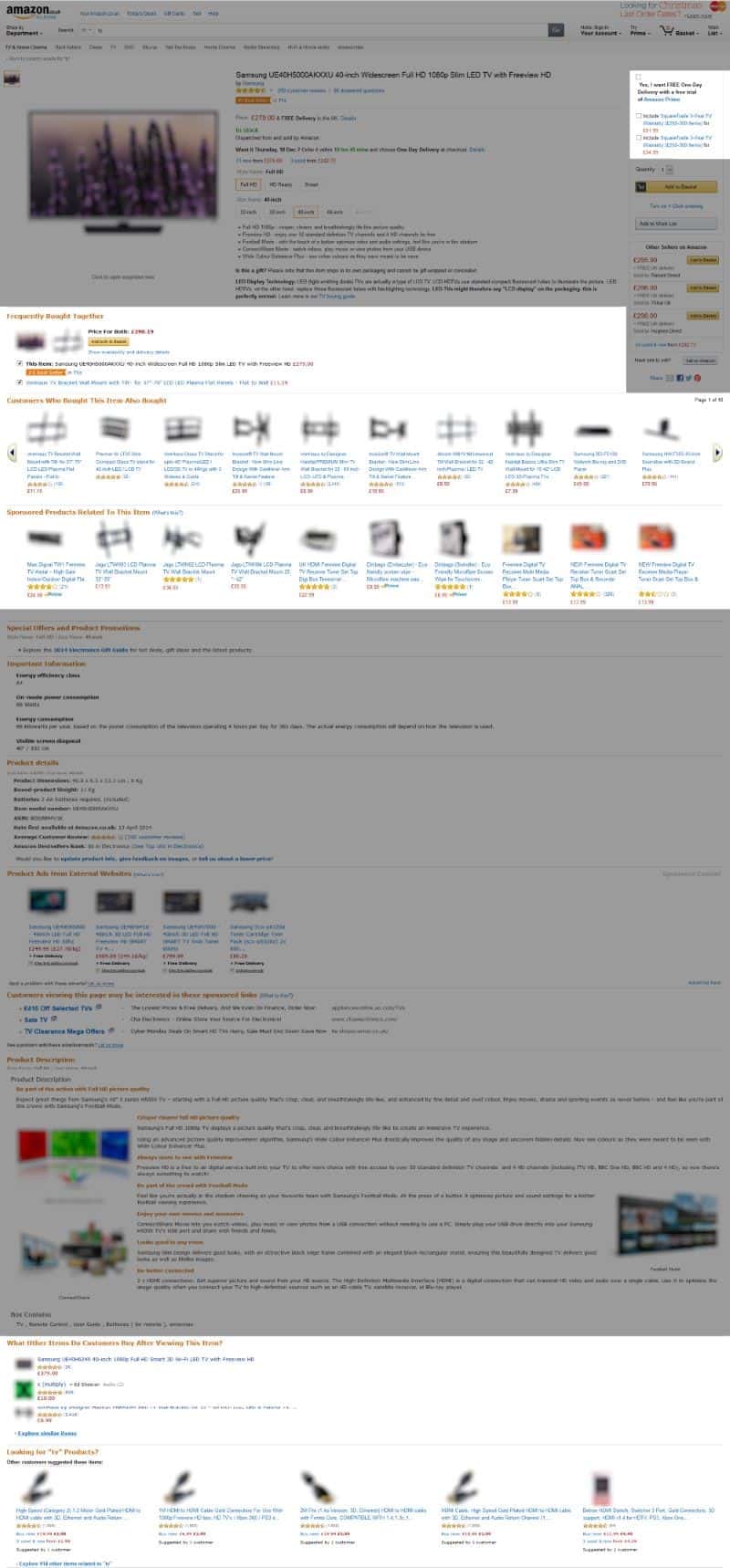This image is a screenshot of an Amazon product page with specific sections highlighted. The darkened background renders most of the page illegible, emphasizing only the focused areas. In the top right, a white box stands out, but the black text at the top is too blurred to read. Underneath, two checkboxes feature blue text and red prices, both also blurred beyond recognition. Another highlighted section spans horizontally across the page's center top, displaying a series of product thumbnails that are too blurred to discern details. Each product has a blue title, a star rating, and a price listed beneath it. At the bottom of the page, another highlighted section shows a similar array of products, with completely blurred images, blue titles, star ratings, and red prices against a white background. Despite the overall blurriness, it is possible to make out an image on the top left of a computer monitor displaying purple flowers, accompanied by the product title "Samsung 40-inch widescreen Full HD 1080p, 58-centimeter LED TV with Freeview HD."